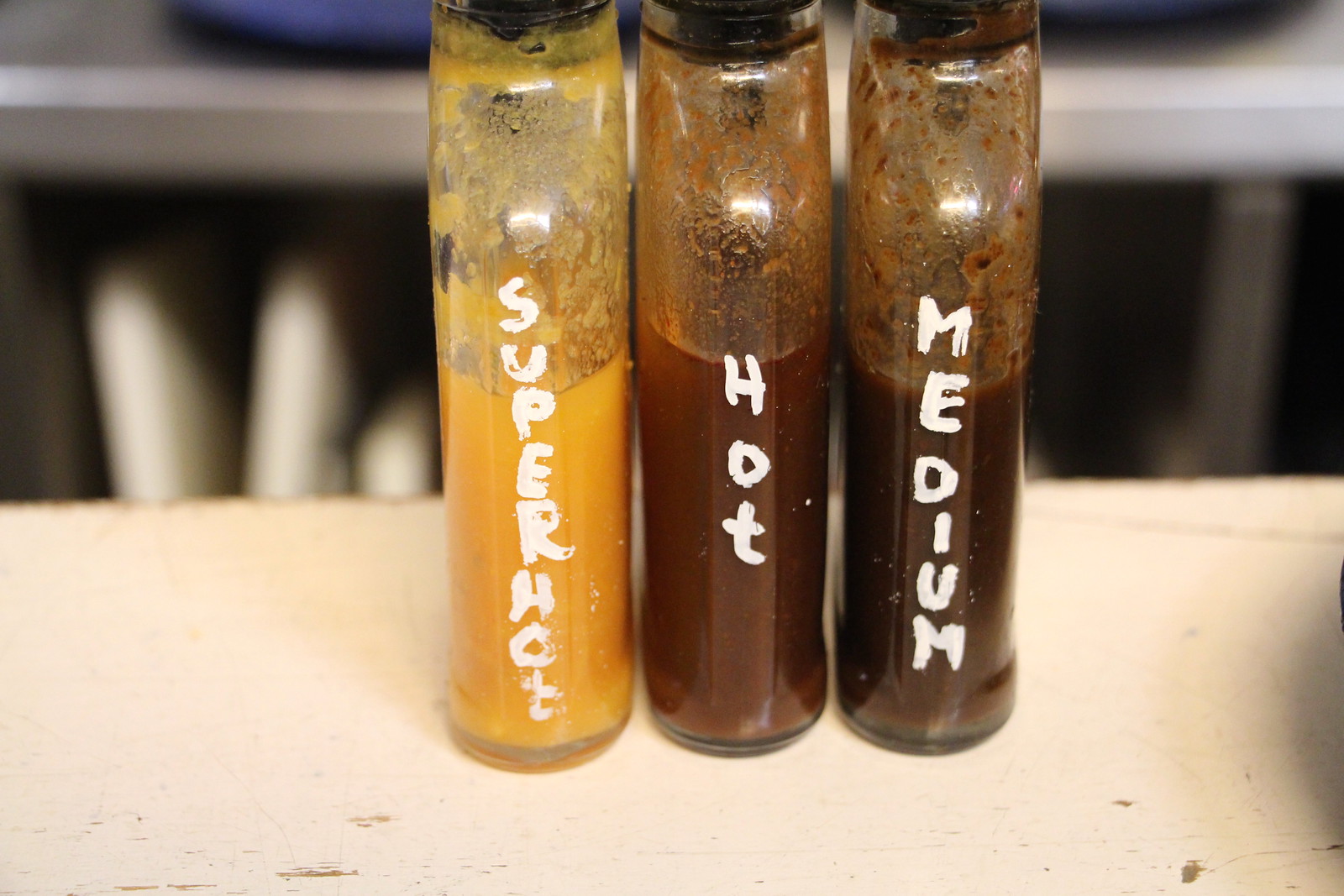The image depicts three partly used bottles of barbecue sauce arranged side by side on a white, slightly worn wooden table. Each of the transparent bottles, showing residue at the tops, bears a different label printed vertically in white text: "Super Hot," "Hot," and "Medium." The "Super Hot" sauce in the left bottle appears yellow-orange, the middle "Hot" sauce is red, and the "Medium" sauce in the right bottle is a darker brown. In the background, there is a counter or shelf displaying three upright white plates in a holder. The scene is captured from a side angle, highlighting the thickness and transparency of the bottles.